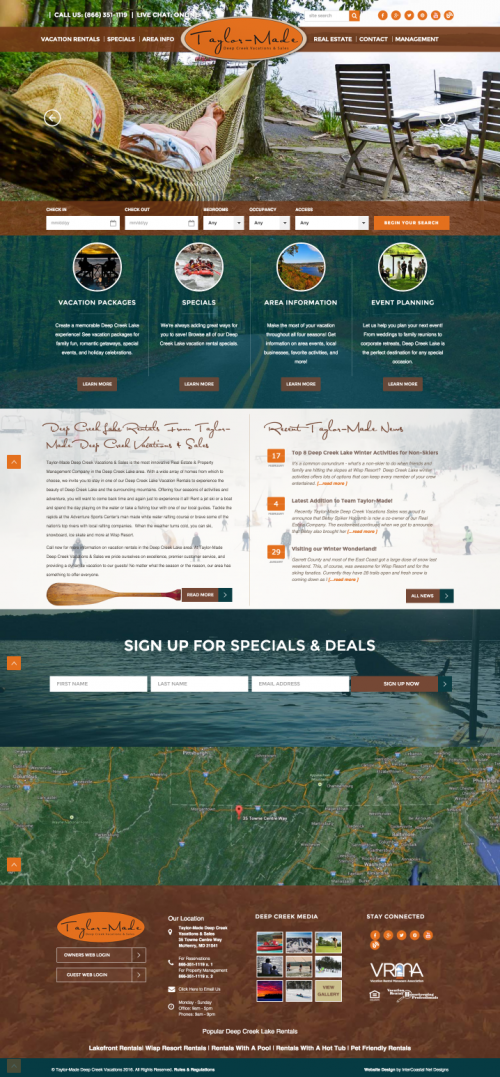The image is a detailed flyer for what appears to be a vacation rental service or travel agency. The top section of the flyer features a set of small, easily missed texts, with some descriptive pictures above them. Among these, there is a relaxing visual of someone lounging in a hammock, evoking a sense of tranquility and leisure. Beside this image is an orange logo with the brand name "TaylorMade."

At the very top of the page, you can find navigational links labeled "Vacation Rentals," "Specials," "Area Info," "Real Estate," and "Contact Management," accompanied by various social media icons for wider audience engagement.

Below these links, there are search boxes designed for users to input their check-in and check-out dates, alongside a prominent "Begin Your Search" button to streamline the rental searching process. Following this section, the flyer showcases four thematic images: the first illustrating vacation packages, the second depicting specials, the third providing area information, and the fourth focusing on event planning. Each of these images is complemented with brief captions that, though hard to read, add to their descriptive nature.

Towards the bottom of the flyer, there is a map indicating a particular location, though the specifics are unclear. Nearby, there is a sign-up section for special deals with search boxes, enhancing user engagement and interaction. A vivid image of a dog joyfully jumping into a large body of water serves as the flyer’s eye-catching backdrop, reinforcing a sense of adventure and fun.

The footer of the flyer repeats the "TaylorMade" logo in orange and includes several links along with additional social media icons. The color palette used throughout the flyer integrates earthy tones of brown with white, orange, and green, providing a harmonious blend that resonates with nature and adventure. Various sections of the flyer feature orange buttons and brown or nature-themed backgrounds, enhancing its visual appeal.